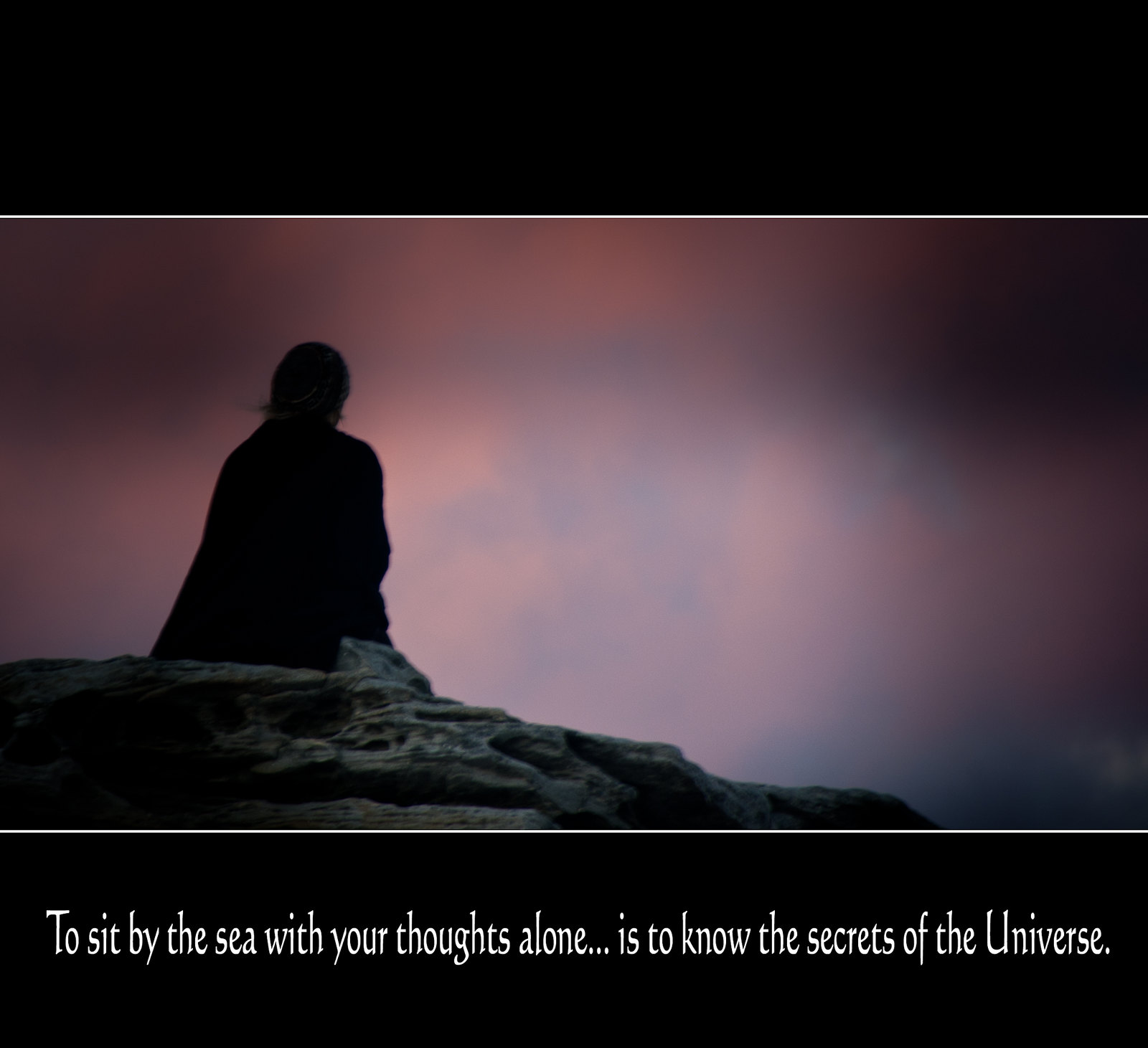The image is a color photograph framed by a thick black border both at the top and bottom, with an inner white border framing the central photograph. Within the bottom black border, white text reads, "To sit by the sea with your thoughts alone is to know the secrets of the universe." The photograph depicts a rocky outcrop with a silhouette of a person sitting on the rocks, looking outward. They are wearing long-sleeve clothing, making their specific features indistinguishable due to shadows. The sky above them is a gradient of blue, pink, and white, suggesting either a sunset or sunrise. The contemplative scene is captured such that no sea is visible, focusing solely on the sky and the person's silhouette.